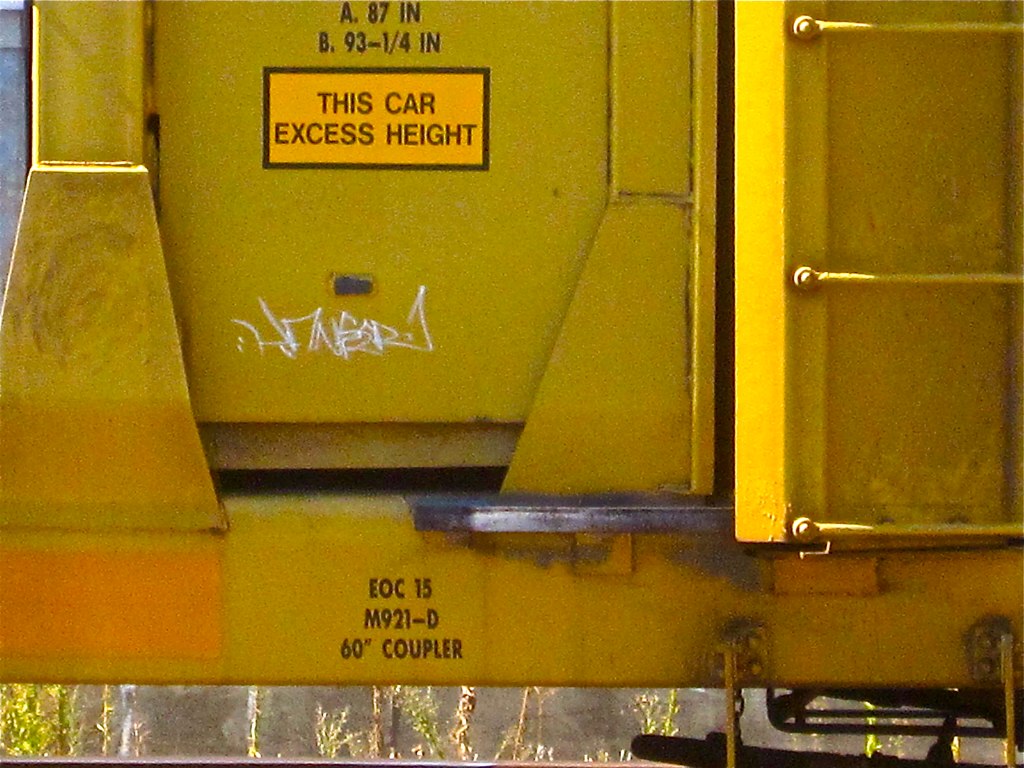This detailed photograph showcases the yellow side of a freight train car, partially covered in dirt and grease. The car is elevated, revealing grass and weeds growing underneath. On the left side of the image, there is a slender metal column that widens slightly at the bottom, and a thick metal bar runs horizontally above the exposed ground. The yellow surface features numerous inscriptions: at the top, it reads "A 87 IN" and "B 93 1 1⁄4 inches" in black text. A prominent yellow rectangle with a black border, located slightly lower, declares "This Car Excess Height" in bold black font. Below this rectangle, there is white graffiti or chalk scribbling. Further down, just above a gray metal step, the text "EOC-15 M921-D 60 inch coupler" is displayed in black. On the right side, there is a ladder composed of three thick metal rungs extending off the frame. The top left corner of the photograph reveals a small patch of concrete, contributing to the gritty, industrial atmosphere of the scene.